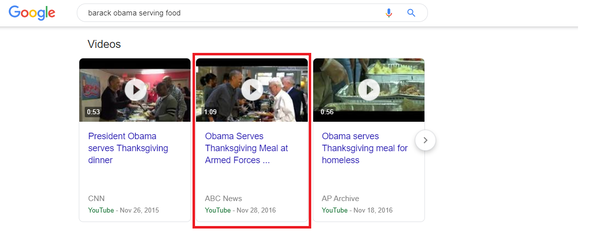The image displays search results on Google for videos of Barack Obama serving food. There are three video thumbnails. The first video, which is 53 seconds long, shows President Obama standing and serving food to a room filled with people in a cafeteria-style setting. In the second thumbnail, President Obama is depicted in a different location, distinguished by different attire and the presence of windows; this video also revolves around him serving Thanksgiving meals. The final video, lasting 56 seconds, is titled "Obama serves Thanksgiving meal for homeless" and features tin foil pans filled with food. All the videos capture different instances of President Obama engaging in acts of service, including serving meals to the armed forces, the homeless, and participants in a dinner event.